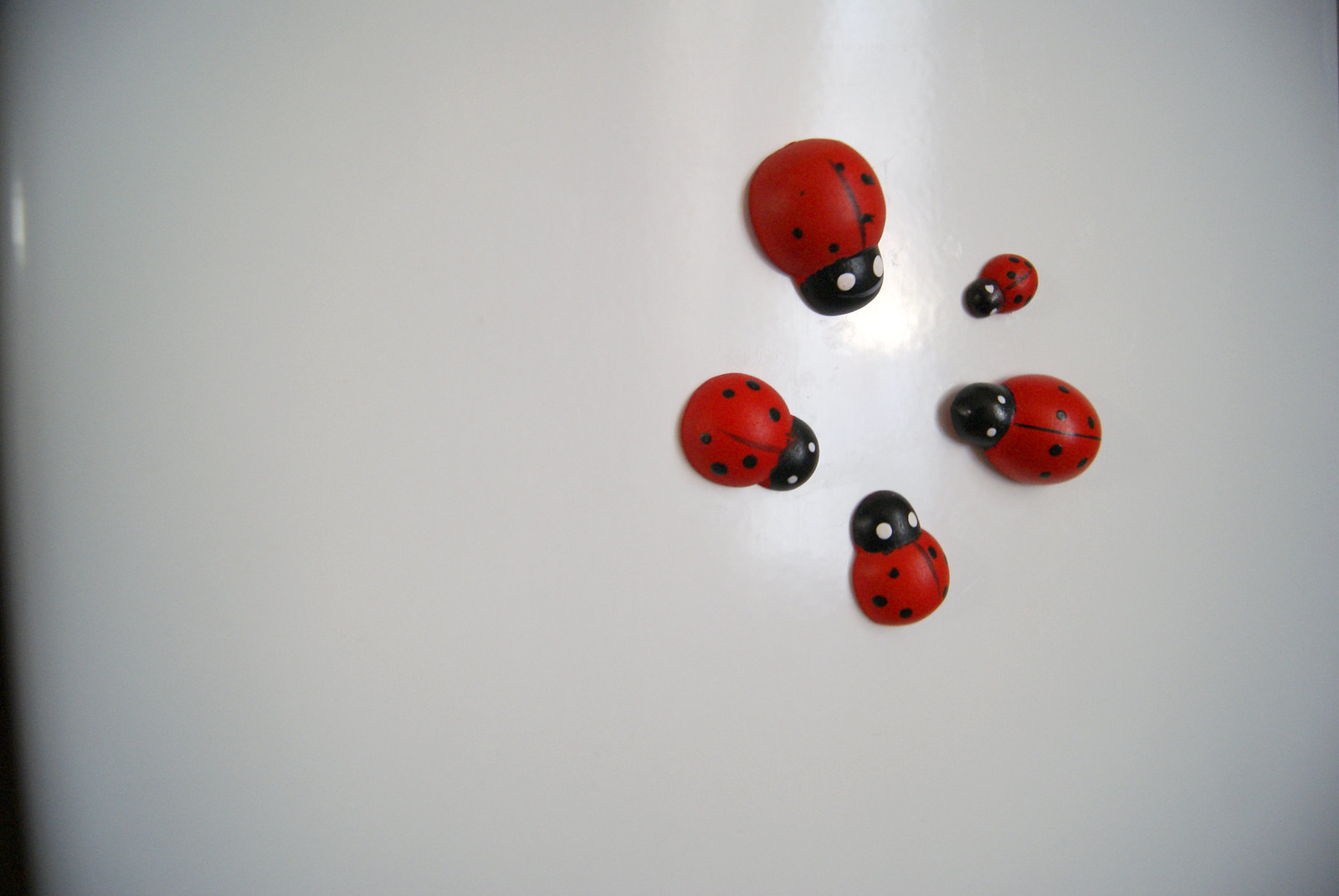The image is a close-up photograph of the front of a glossy white refrigerator with five plastic ladybug magnets arranged in a circle. The ladybugs are distinctively designed with black heads featuring two white eyes, a black line down the center of their red bodies, and three black spots on either side of the line forming a triangular pattern. The largest ladybug is at the top and faces downward, about four times the size of the smallest ladybug, which is positioned in the upper right-hand part of the circle. The arrangement follows a pattern of largest, tiny, medium, small, then medium again in a clockwise formation. The surface of the refrigerator is clean and reflective, adding to the vividness of the colors and details. Some ladybugs exhibit wear, particularly on the central line, adding character to the scene.